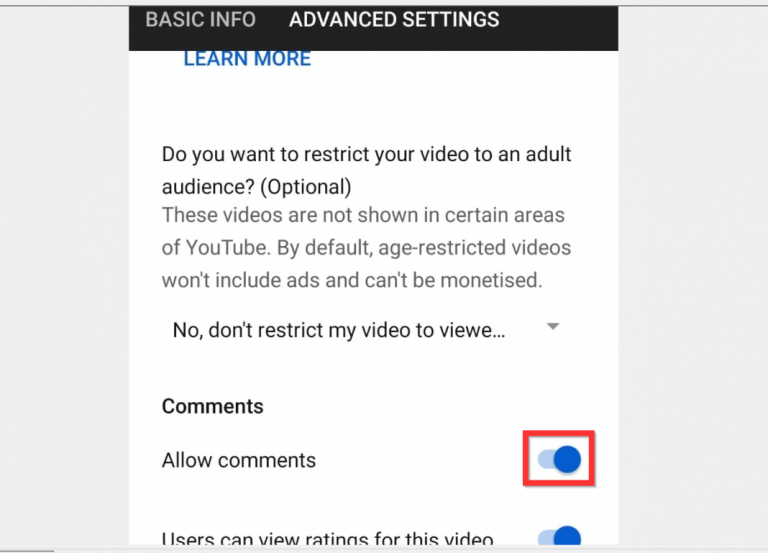The image showcases a website interface, seemingly from a video platform like YouTube. At the top, there is a black navigation bar. Within this bar, the text "Basic Info" appears in gray, while "Advanced Settings" is highlighted in white. Directly below, a section asks, "Do you want to restrict your video to an adult audience?" with an indication that it is optional. Above this question, there is a "Learn more" link that users can click for additional information. The information provided states, "These videos are not shown in certain areas of YouTube. By default, age-restricted videos won't include ads and can't be monetized."

Further down, there is an option labeled "No, don’t restrict my video to viewers over 18," accompanied by a drop-down arrow for additional choices. In the comments section, the interface shows the option "Allow comments." There is a conspicuous red box with a large blue illuminated circle inside, featuring a light blue slider cut, indicating an active selection. Additionally, the setting "Users can view ratings for this video" is also enabled, as indicated by another large blue circle that is switched on.

Above all these settings, "Learn more" links are available for additional context. The top border of the website features a line that traverses the entire width, though there is an unconnected segment originating about one-eighth from the left-hand side.